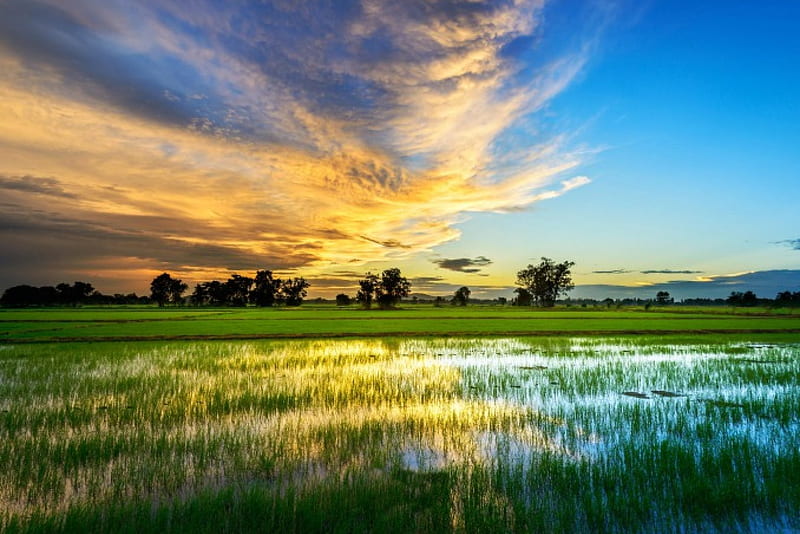This mesmerizing photograph captures a serene, grassy marsh at the end of the day, reflecting the warm hues of the sun in its waters. At the horizon, a lush green field meets a scattering of silhouetted trees, marking the transition between land and sky. In the background, the right-hand side reveals distant mountains or hills beneath a clear blue sky, gently blending with hints of white at the horizon. The left side of the sky is adorned with wispy cirrus clouds, their bottoms illuminated in a yellowish-brown hue, contrasting against their white and gray tops. In the foreground, the flooded marsh resembles a rice paddy, with stalks of grass protruding from the water, adding intricate detail to this peaceful landscape.